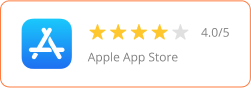In this image, we are looking at a basic screenshot set against a completely white background. At the top of the screenshot, encased in a thin yellow border, there is a horizontally elongated rectangle. On the left side of this rectangle, a blue box contains the letter "A." To its right, a four-out-of-five star rating is displayed prominently. Adjacent to the star rating, gray text reads "4.0/5." Below this rating, in smaller gray text, the words "Apple App Store" are clearly visible.